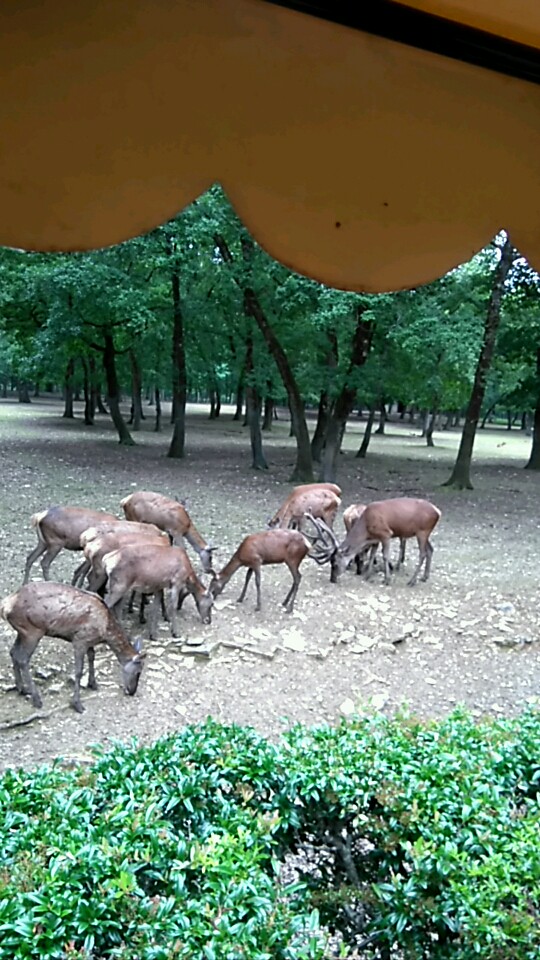In the center of the bright daytime photograph, a herd of roughly 10 to 13 deer grazes on a predominantly gray dirt field. The deer are a mix of dark brown and reddish-brown shades, with white rumps and varying sizes, indicating both adults and juveniles. One prominent stag with a substantial set of antlers is located on the right-hand side of the image, facing left. The majority of the deer are shown in profile, their heads bent down as they feed, with most facing to the right.

The foreground features a thick, neatly trimmed green hedge running across the bottom of the image. The background reveals a sparsely populated orchard-like area with mature trees, and the grass there appears well-manicured. The upper portion of the image includes a scalloped canopy edge, possibly from an awning or patio umbrella, suggesting the photo may have been taken from a porch. The image is well-focused, vibrant, and devoid of any text or print.